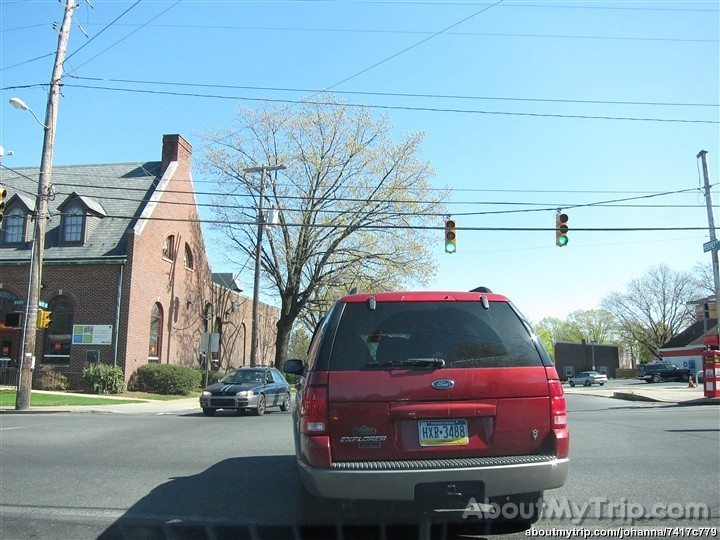This is a detailed color photograph taken from the point of view of someone sitting inside a car at a road intersection. Prominently in the foreground, directly ahead, a red Ford Explorer with black-tinted windows and license plate AXRHXR.3488 can be seen. The intersection is active, with another small black car making a right turn in front of a red-bricked church visible in the background.

The intersection features traffic lights, currently green, which are suspended from wires crossing overhead, attached to poles. The bright blue sky above is mostly clear, with only a few diffused clouds near the horizon. The scene also includes various urban elements; buildings, lighting poles, telephone wires, trees, and even a post office can all be spotted in the surrounding area.

Adding a touch of personalization, there is a watermark text at the bottom right corner of the photograph that reads "aboutmytrip.com/about/my/trip.com/forward/slash/johanna/7417c779."